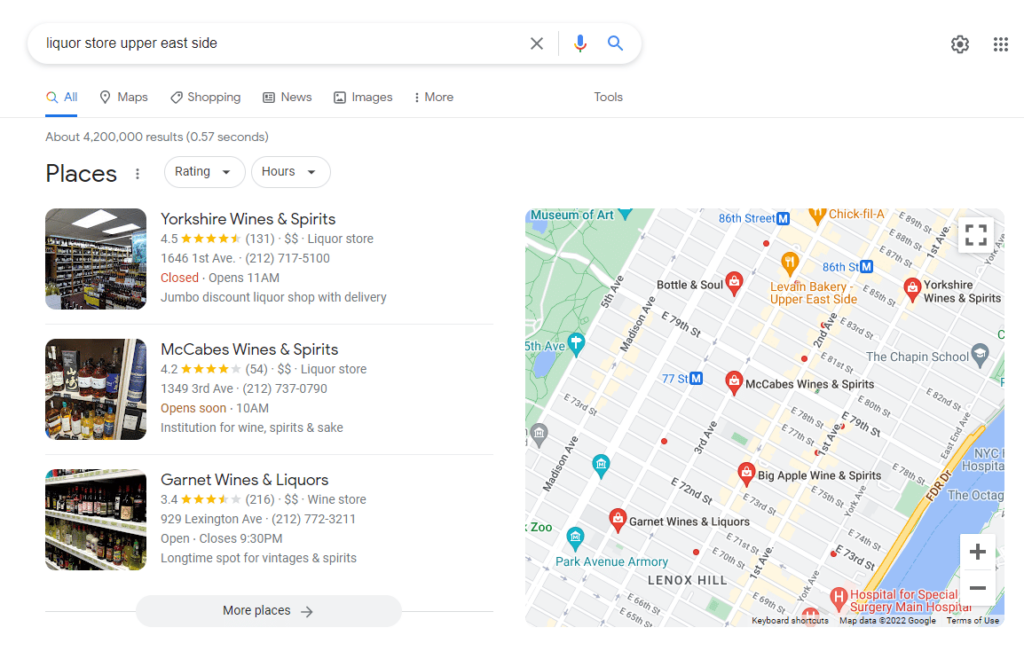This image shows a Google search result for liquor stores on the Upper East Side of New York City. On the right side, there's a detailed map peppered with at least five points of interest, prominently featuring the nearby body of water, the FDR Drive, and cultural landmarks like the Metropolitan Museum of Art. Visible businesses on the map include Chick-fil-A and a local bakery. On the left side, the search results list several liquor stores:

1. Yorkshire Wines and Spirits, rated 4.5 stars.
2. McCabe's Wine and Spirits, with a 4.2-star rating.
3. Garnet Wines and Liquors, rated 3.4 stars.

Each listing indicates a moderate price range with two dollar signs ($$) and features store photos, mostly showing rows of wine shelves. The interface is simple, with a white background and occasional blue accents. The map also displays numerous numbered streets like 79th and 72nd. Below the listings, there's a "More Places" button for additional results.